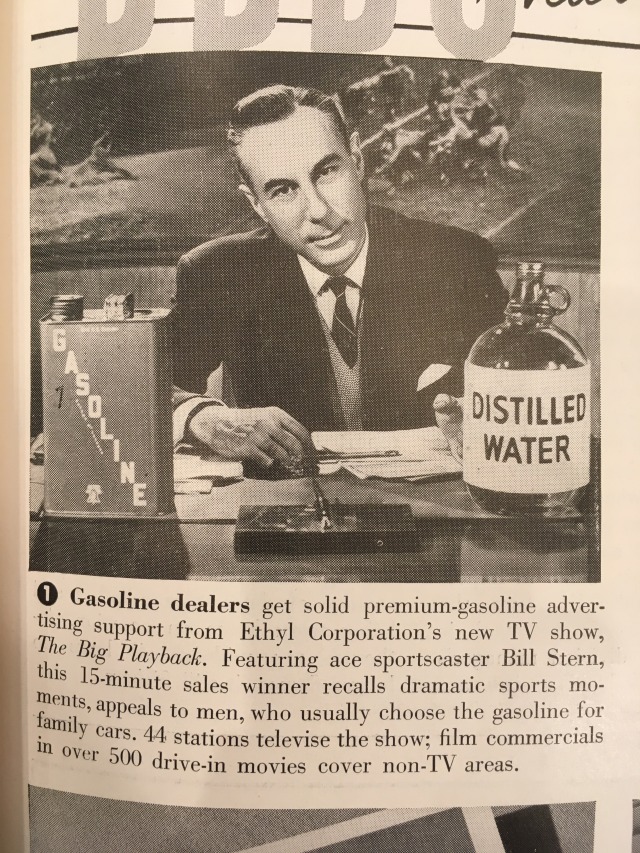The image is a slightly convex, sepia-toned newspaper clipping, suggesting an aged artifact, not laying entirely flat, with edges of other articles visible at the top and bottom. The main focal point is a smartly dressed man with slicked-back hair, wearing a tie and a pocket square, sitting at a desk and facing the camera. At his left on the desk is a gasoline can labeled "gasoline" diagonally in white text, and at his right is a laboratory-style jar marked "distilled water" in black text. An ink quill is also positioned at the front of the desk. Below the image, a caption reads: "1. Gasoline dealers get solid premium gasoline advertising support from Ethel Corporation's new TV show, 'The Big Playbook.' Featuring ace sportscaster Bill Stern, this 15-minute sales winner recalls dramatic sports moments, appeals to men who usually choose the gasoline for family cars. 44 stations televised show; film commercials in over 500 drive-in movies cover non-TV areas." The advertisement is likely from the 1930s or 1940s, reflecting the era's marketing techniques and media landscape.